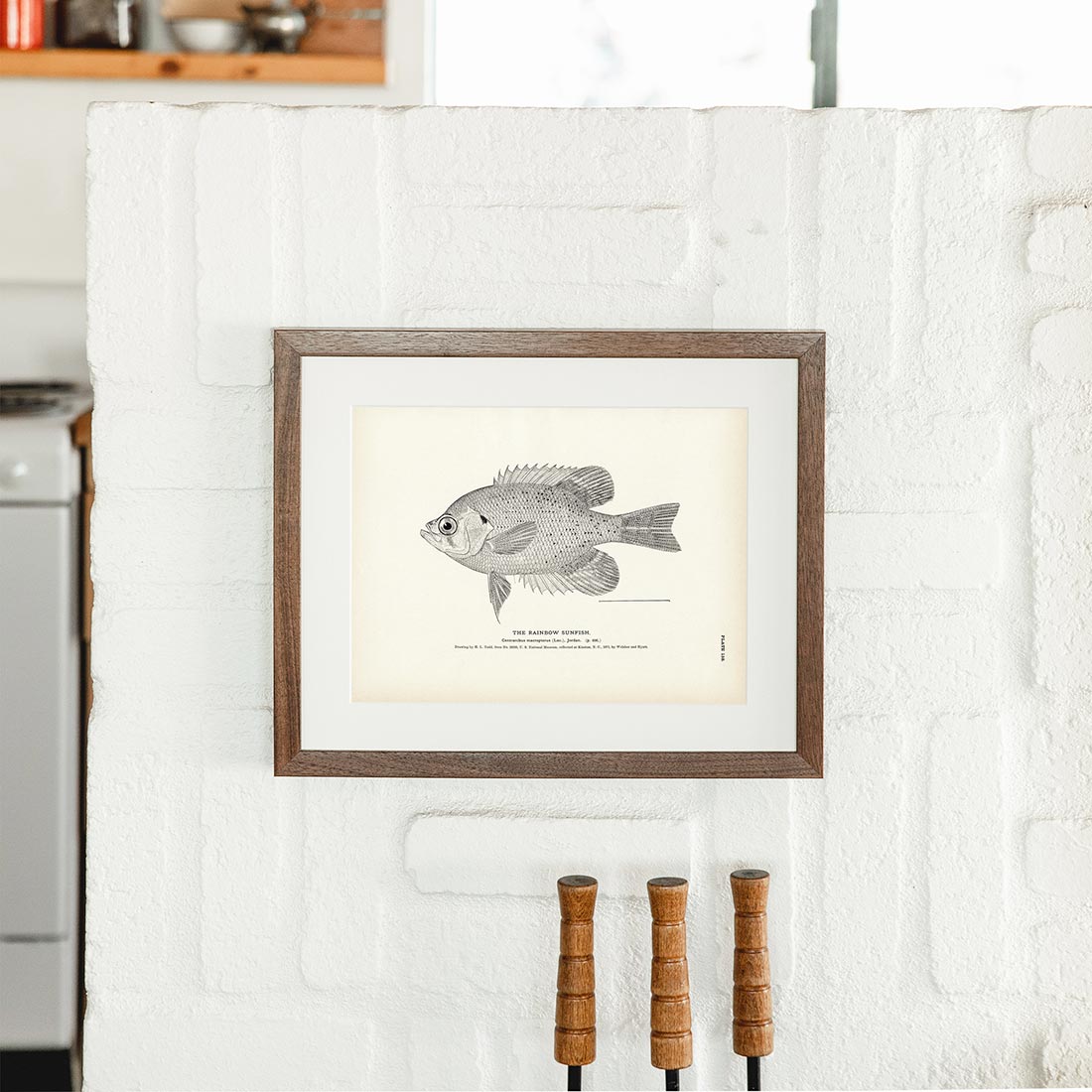The image showcases a black and white illustration of a fish, specifically a rainbow sunfish, against what appears to be a light green, almost velvet-like background, though some might describe it as aged yellow. The fish, depicted in profile and looking to the left, has a notably shaded gray face, a protruding bottom lip, and a distinctive oval eye with a black dot in the center. It features large spiked fins on both the top and bottom, and additional fins extending from its body and tail. The illustration is encased within a white matting, bordered by a brown wooden frame. Beneath the fish, there is tiny black text identifying it and some additional smaller, illegible writing. The framed artwork hangs on a roughly textured, white-painted brick wall. Below the frame, three wooden handles with wrought iron poles are visible, suggesting items like fireplace pokers. The left side of the background reveals a hint of a kitchen, including part of a stove, a shelf, and a window above.